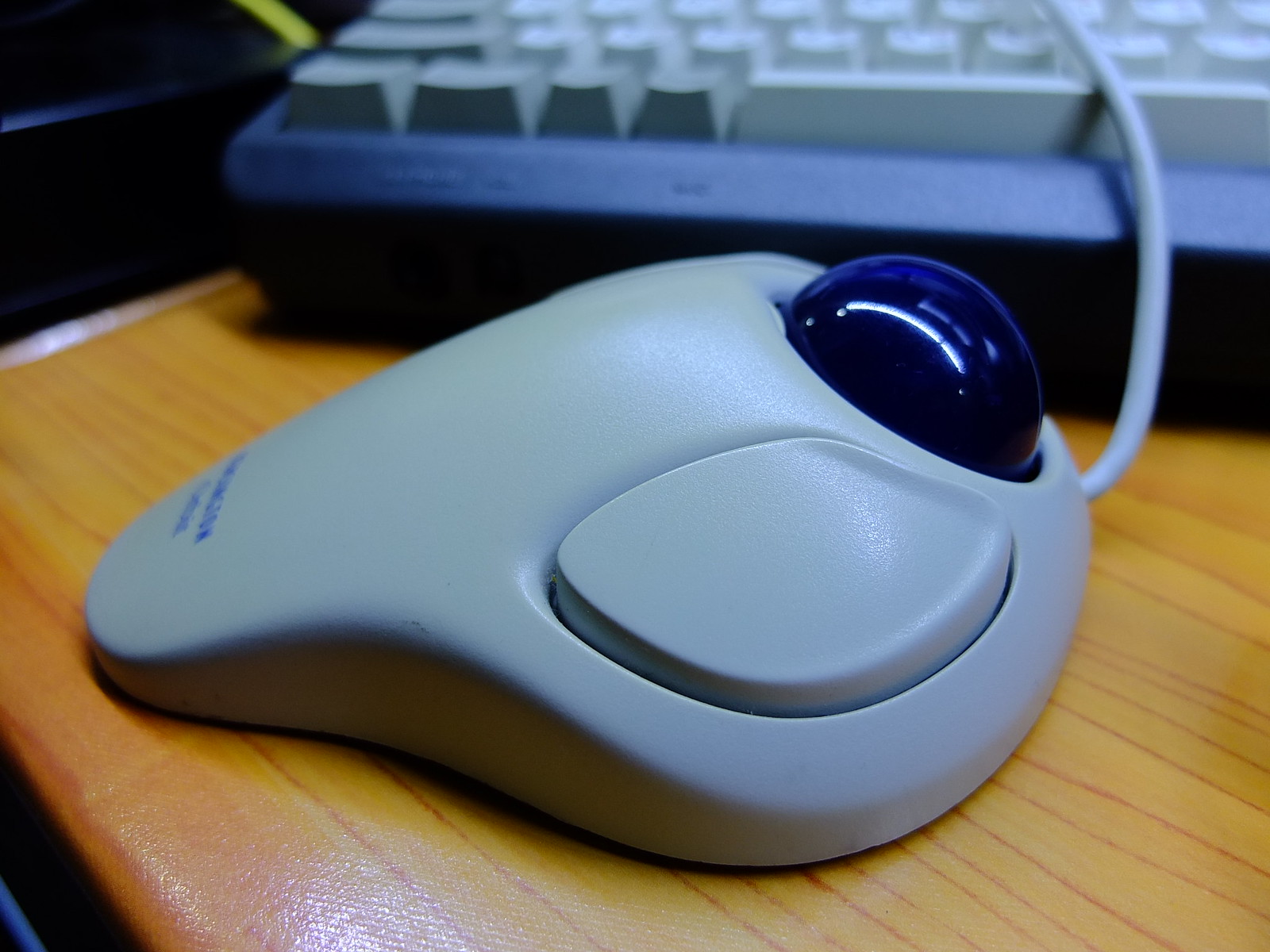This detailed photo, taken indoors, features a close-up of an old-school 90s-style gray trackball mouse. The mouse, uniquely shaped almost like an alien head, is positioned with its large black trackball pointed to the right. We can see the single, prominent button to the side of the trackball. Below the mouse, the light tan, yellowish desk or pad, with its wood-like texture and dark burnt orange grain, provides a striking background.

In the photograph's blurred background, an old-style keyboard with a blue casing and gray keys is partially visible. At the top left corner, there is a faint, indistinct blue and yellow object. The mouse's wire is seen trailing upwards and resting on the keyboard, creating a nostalgic tableau of retro computing peripherals.